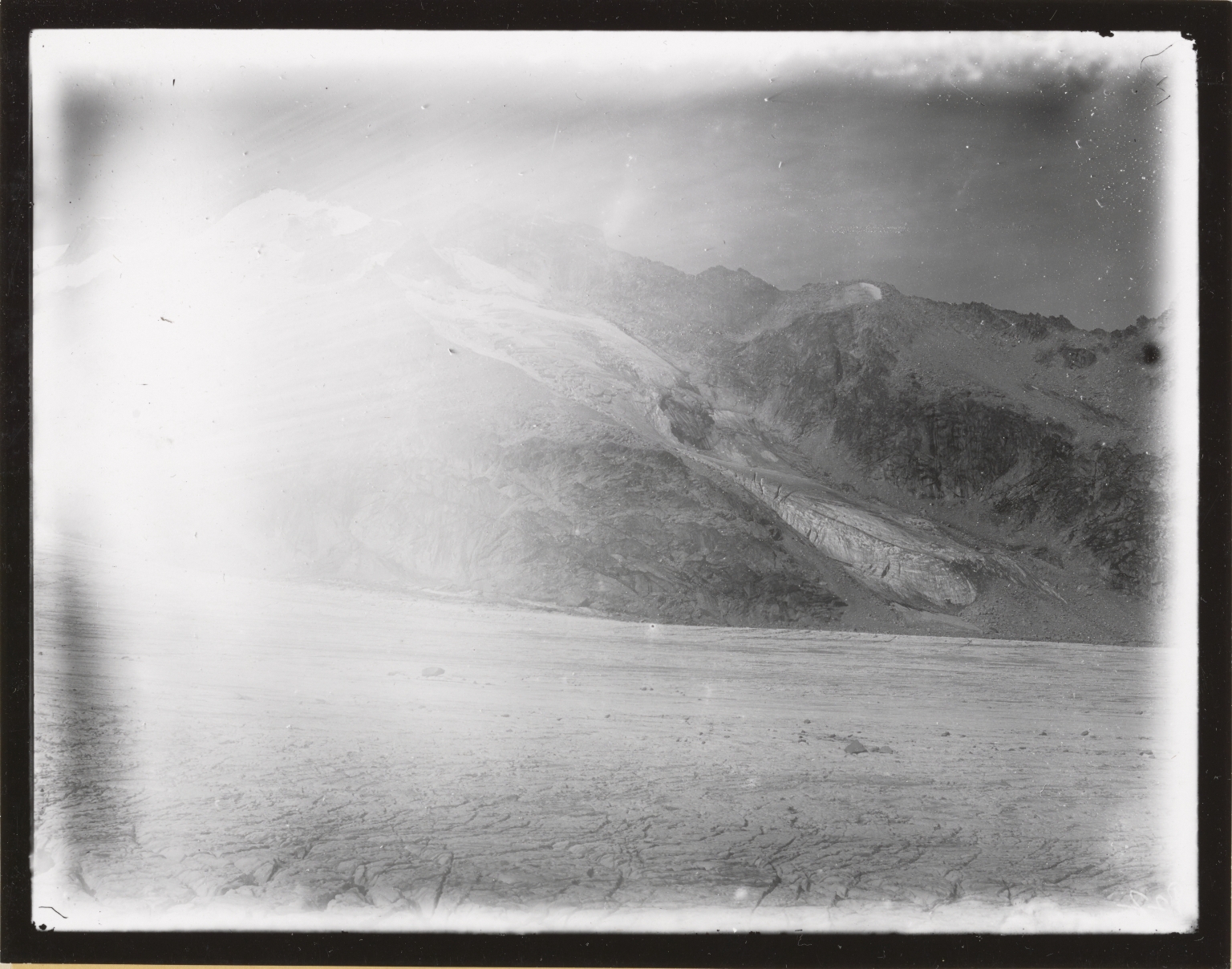The image is an old, faded black and white photograph, possibly deteriorated or intentionally styled for an aged effect. It features a rugged, mountainous landscape with a distinct hillside or mountain range rising prominently on the right side of the frame. In the foreground, the ground appears broken and cracked, evoking the look of mud flats or possibly a glacier, laced with dark fissures. The left side of the image is heavily whited out, possibly due to damage or intentional glare akin to bright fog or sun exposure, giving the appearance of a giant cloud. The sky above is lightly marked with cirrus clouds, suggesting it was a somewhat cloudy day. The photograph is bordered by a black trim, adding to its vintage aesthetic. This detailed portrayal captures the serene and stark beauty of the landscape, emphasizing its age and weathered charm.